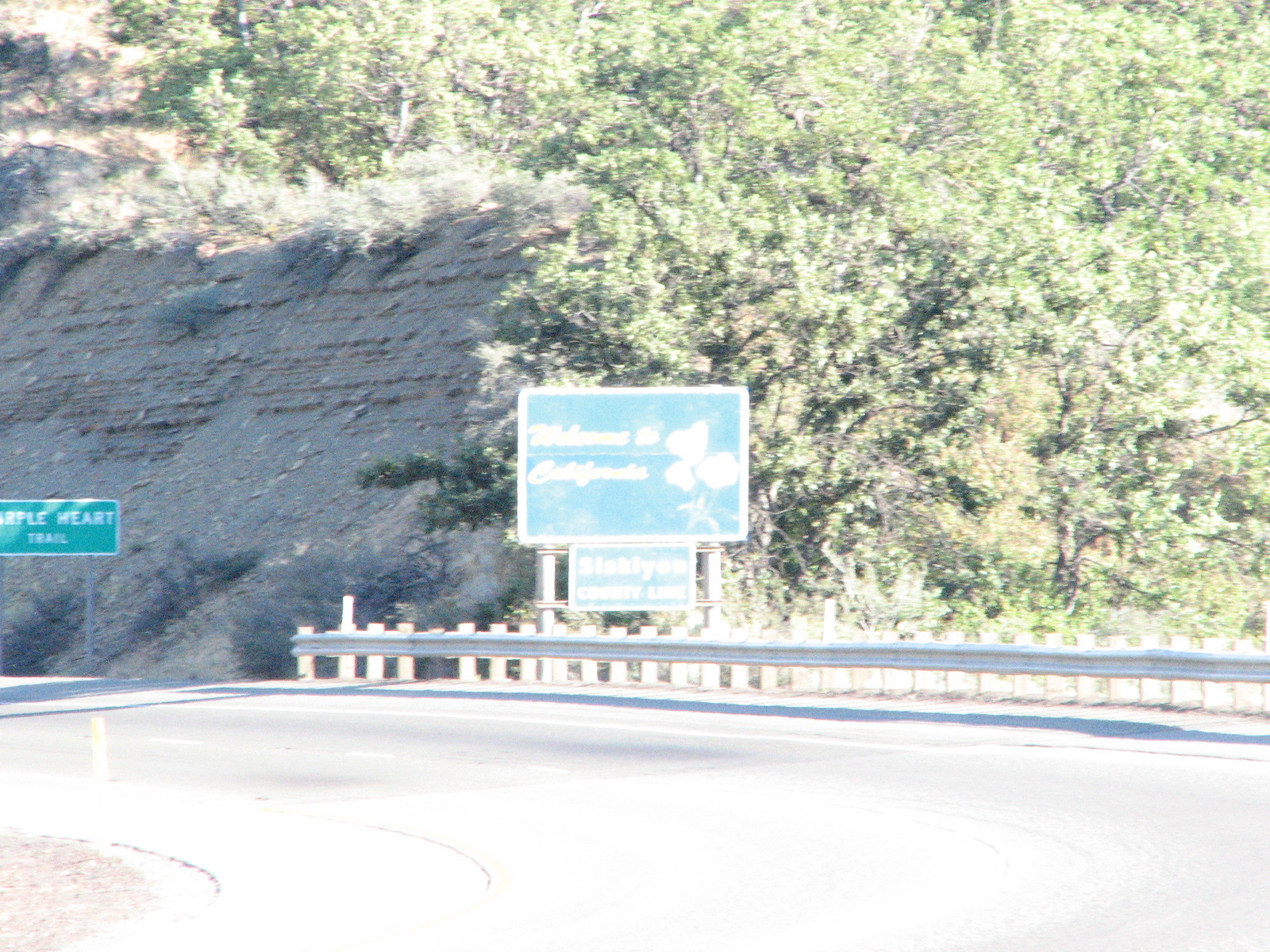This photograph captures a curved section of a highway road bordered by a silver guardrail on the far side. The road, situated on a mountain, is flanked by a steep, rocky face composed of slate and reaching approximately 20 to 30 feet high. This rocky face transitions into brown grass and dense, leafy deciduous trees that extend upwards, covering most of the mountain slope. Toward the left side of the image, the road features two green signs, one of which is partially illegible due to sun glare but suggests 'Maple Heart Trail,' and the other welcoming travelers to California. Additionally, some bushes and greenery are scattered along the base of the rocky face next to the road, completing this scenic and winding mountain highway vista.